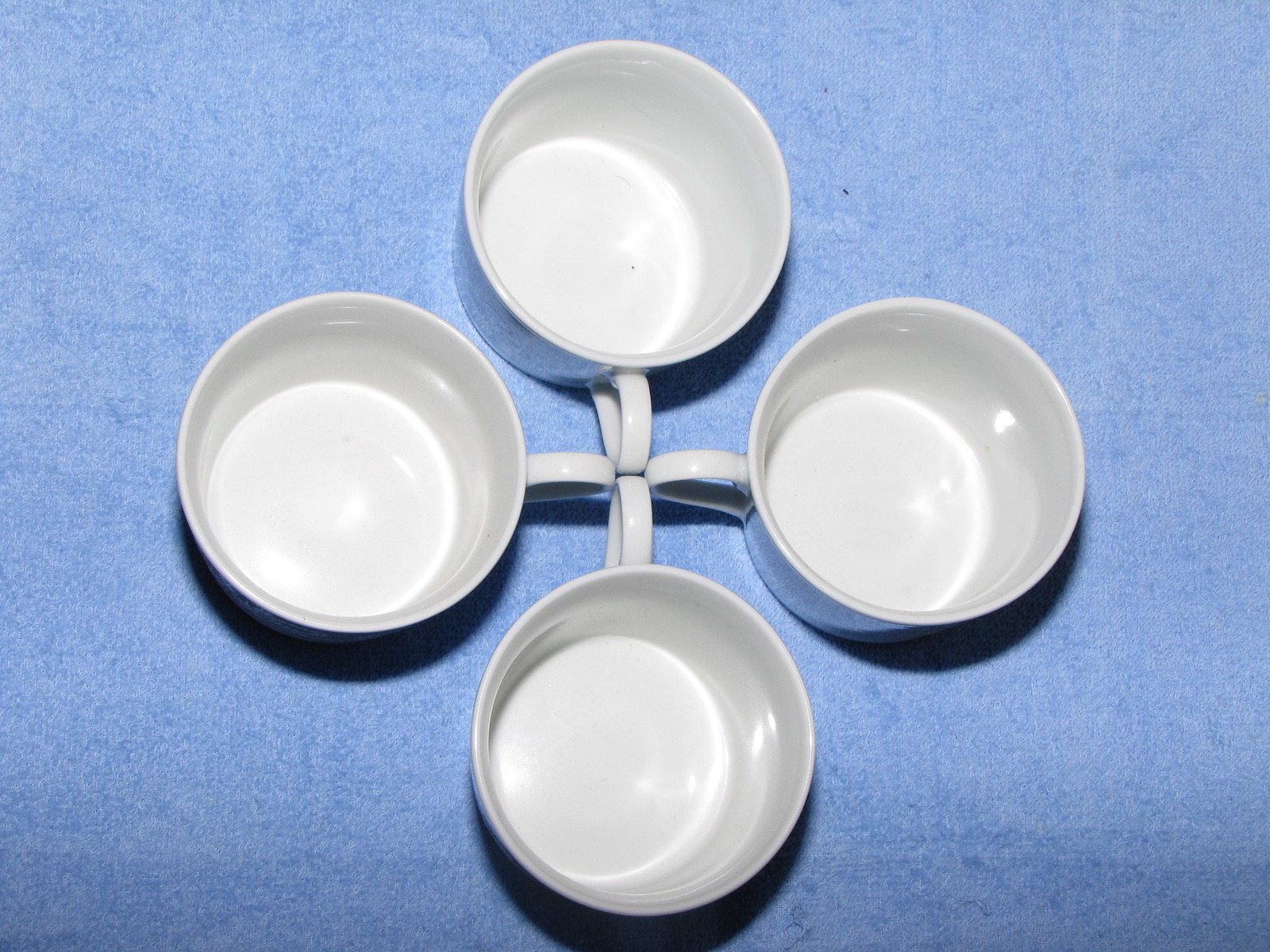The photograph features four white cups arranged in a cross shape on a light blue, fabric tablecloth background. The blue fabric appears lighter towards the center of the image, where a flash may have brightened the middle area, and darker around the corners. The cups are designed with curved handles that touch each other at the center of the image. All the cups seem to possibly contain water. Although the insides and handles of the cups are clearly white, the outside color is ambiguous due to a glossy shine, potentially reflecting the blue tablecloth. From the top view provided, much of the cup bodies are obscured, reinforcing their symmetrical handle arrangement as the focal point.